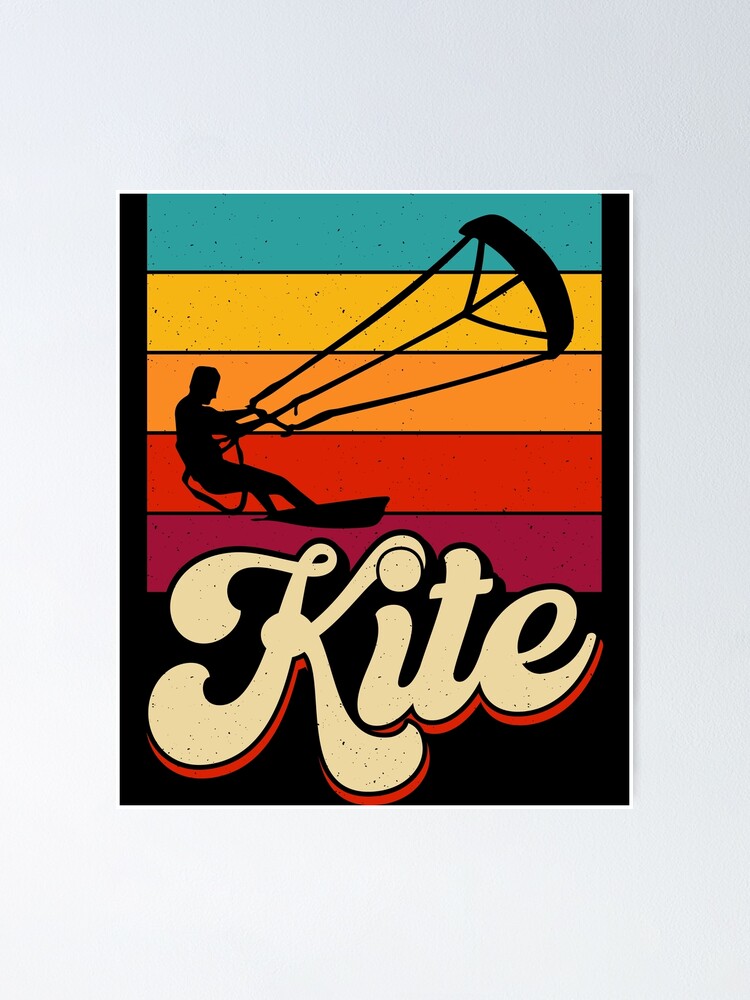This is a vintage-style poster reminiscent of the 1970s, featuring a black background. Vertical stripes in vibrant colors — teal, mustard yellow, orange, red, and maroon — stretch across the poster, forming a striking backdrop. At the forefront, a silhouetted figure engages in a sport akin to kitesurfing or paragliding, depicted with a kite and board in motion over the water. The figure, detailed in black, holds onto the kite, which appears to be billowing with the wind across the scene. Below this dynamic imagery, the word "kite" is prominently displayed in a chunky, brushstroke script font. The off-white lettering is accentuated with a red drop shadow, giving it a bold and stylish appearance.